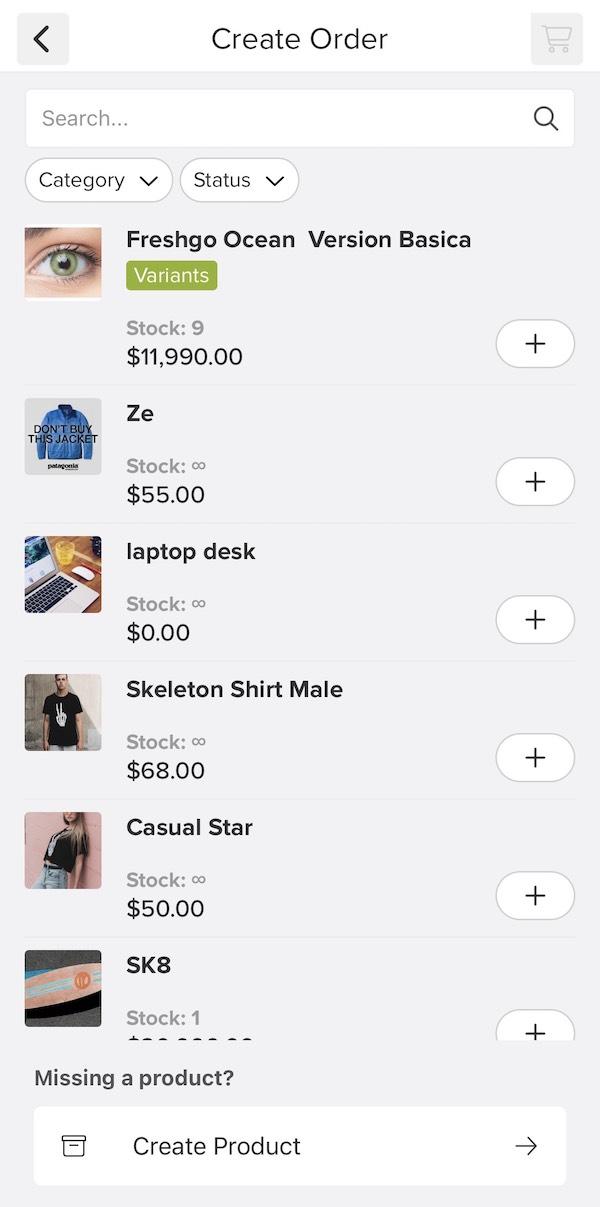A girl wearing a black shirt and jeans leans against a wall. Next to her, there is a brown dildo and various product listings, such as an SK8 skateboard priced at $50 with 1 in stock, a blue coat, a skeleton-themed shirt priced at $68 with infinite stock, a casual star item priced at $50 with infinite stock, and a laptop priced at $0 with infinite stock. The listings also include details about other products and categories, like an $11,990 ZE product with 9 in stock, and a 'Create Order' section, reflecting a shopping cart for various items.